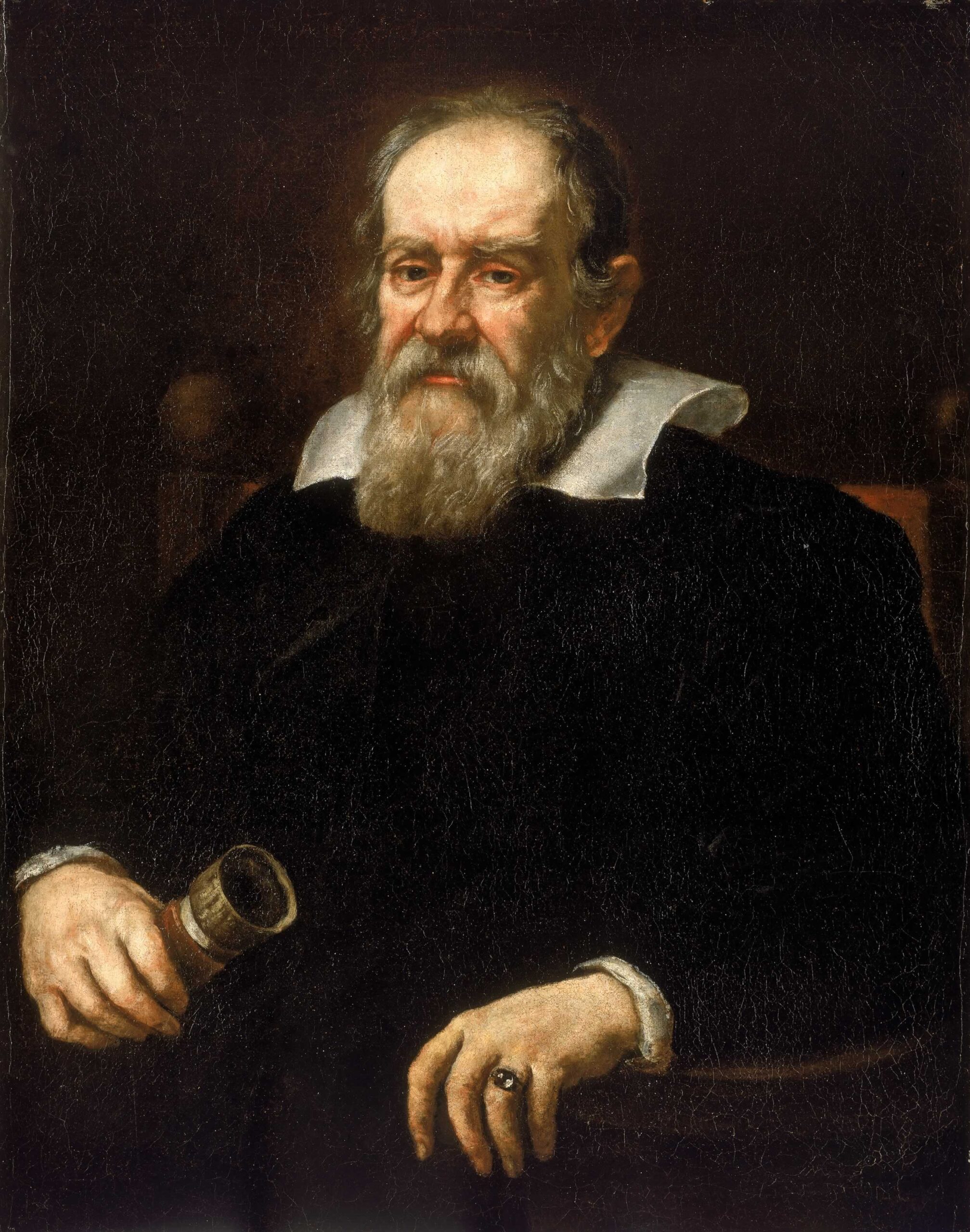This is an old-style portrait painting of an older white man, possibly from the 16th or 17th century, often identified as Galileo. The man is depicted sitting in a large chair with ornate round balls at the top, his right hand resting on the armrest while his left hand holds a circular object—possibly a telescope, reflecting his scientific background, or a scroll. He has a long, gray beard with hints of white, and his hair is similarly graying and receding, indicating age. His attire consists of a long black coat or robe with a white blouse or collar peeking out at the neck and cuffs. He wears a prominent ring on the ring finger of his right hand. The background is a dark, muted brown, which contrasts with the illumination of his stern, somber face and darker eyes. His expression is one of intensity, with arched eyebrows conveying a sense of seriousness and perhaps discontent.